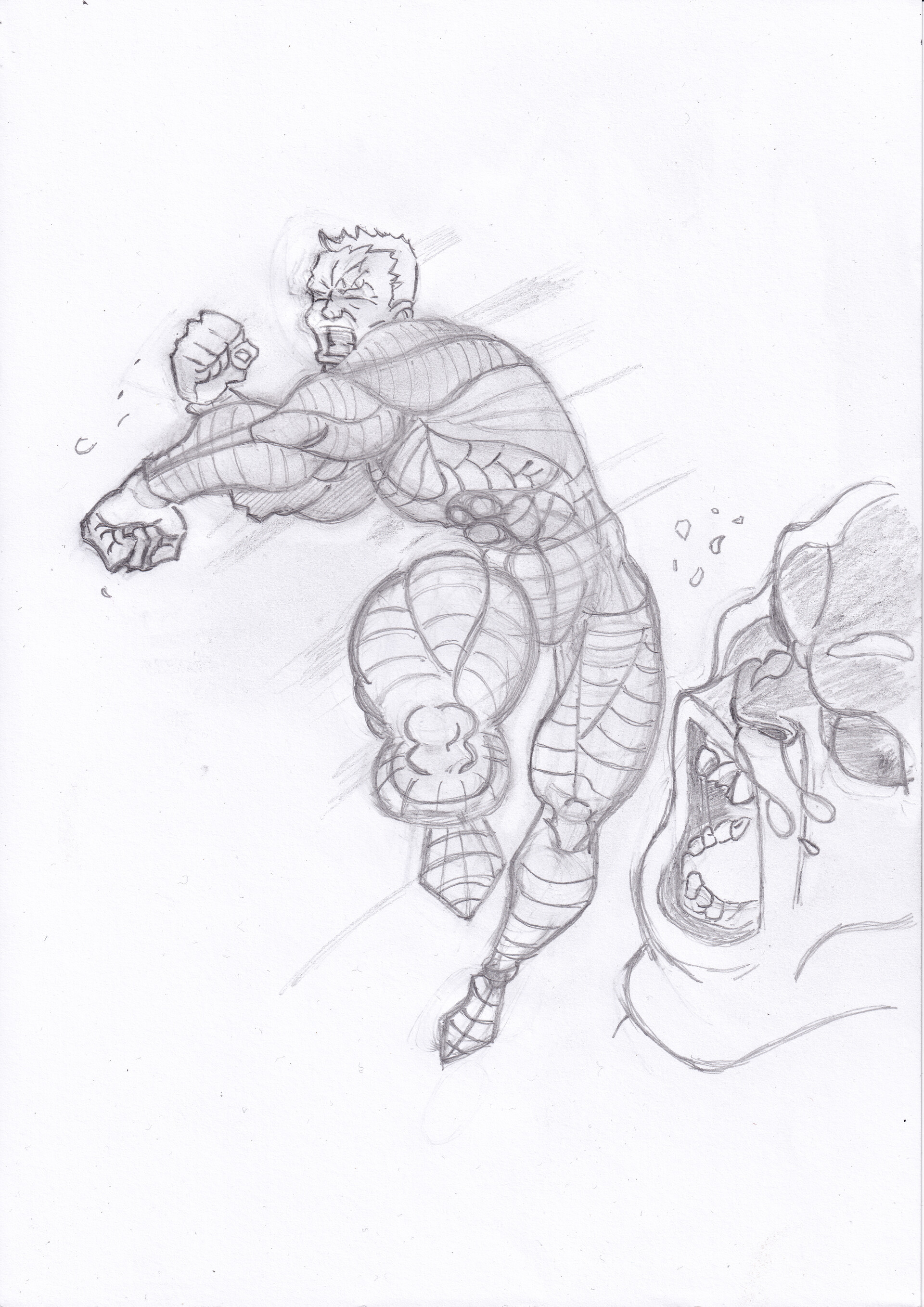The image is a detailed pencil drawing on white paper, featuring a highly muscular superhero with short hair positioned on the left-hand side. The superhero appears to be in mid-action, swinging his clenched fists, with one directed to the right and the other to the left, creating a dynamic fighting pose. His costume is marked with numerous stripes running down his legs and sides, and his veins are prominently visible, emphasizing his bulk and strength. The superhero's facial expression is intense, with his mouth open as if screaming, exuding a fierce determination. 

In the bottom right corner, there is a creature or monstrous figure with a distorted face that has sharp teeth, some of which appear broken, presumably from the superhero's punch. This creature has big black eyes and an open mouth, with what looks like stuff spitting out of its nose, adding to the chaotic scene. The entire drawing, characterized by its shading and intricate detailing, evokes the style of a comic book sketch, capturing a moment of intense action and conflict.